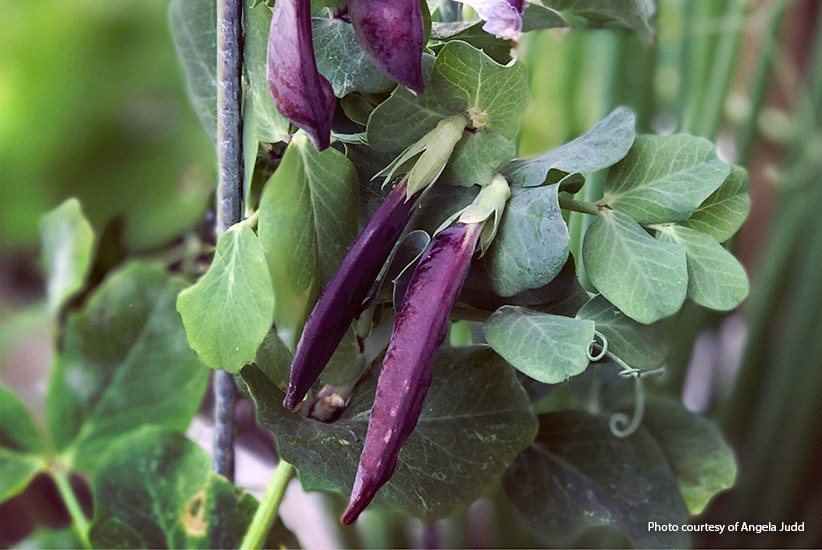This photograph, credited to Angela Judd as noted in white text in the bottom right corner, captures the essence of a unique plant, likely some type of potted legume or bean. The main focus is on the plant's striking purple pods, reminiscent of small eggplants, hanging down like elongated pea pods. These vibrant, eggplant-purple pods stand out against the plant's muted green, oval-shaped leaves, which feature a delicate white veining pattern. The image conveys a sense of recent rain, with tiny droplets visible on the leaves and pods, hinting at the freshness of the scene. In the background, a blur of green vegetation frames the composition, drawing attention to the plant and its four prominent, glossy purple pods, which add a beautiful splash of color to the predominantly green setting. Additionally, some green tendrils can be seen winding through the foliage, complementing the overall natural beauty of this outdoor shot.